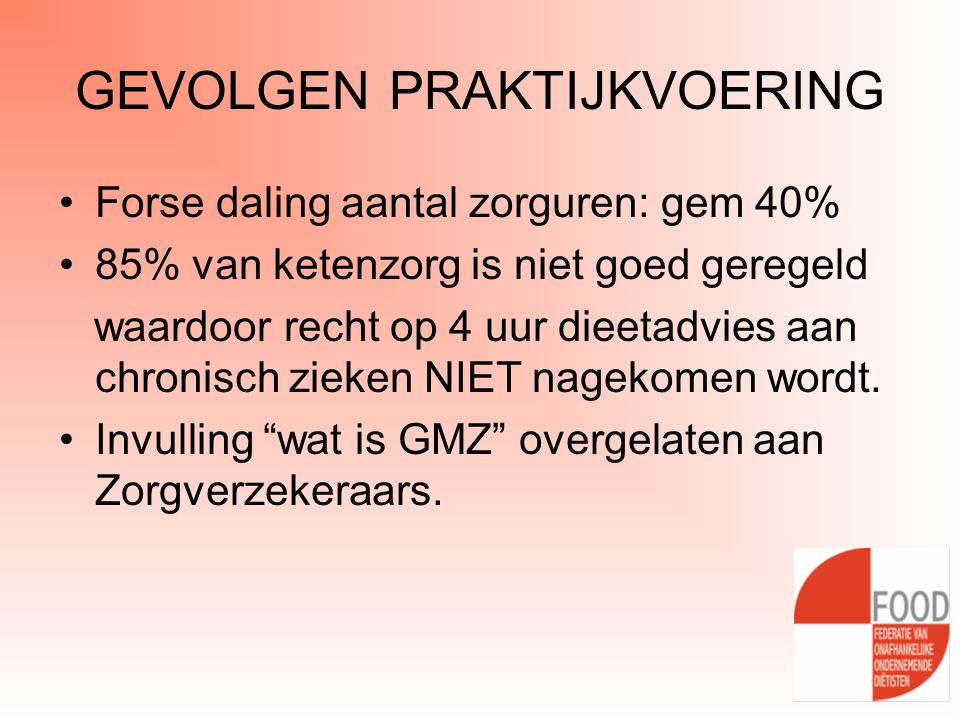This image features a rectangular poster with a fading gradient background, transitioning from a rose or peach color in the top left to white in the bottom right. The top part of the poster prominently displays large, bold, all-capital black text: "GEVOLGEN PRAKTIJKVOERING." Below this, there are three bullet points in black text detailing various percentages and statements: 

1. "FORSE DALING AANTAL ZORGUREN: GEM 40%"
2. "85% VAN KETENZORG IS NIET GOED WAARGED REGELD"
3. "WAARDOOR RECHT OP 4 UUR DIETADVIES AAN CHRONISCH ZIEKEN NIET NAGEKOMEN WORDT."
4. "INVULLING 'WAT IS GMZ' OVERGELATEN AAN ZORGBERZEKERAARS."

In the lower right corner, a white square contains a circular logo divided into red and white quadrants, with the word "FOOD" displayed prominently in gray capital letters within the red quadrants. The design and text elements merge into the faded background towards the bottom and right of the image, giving the overall poster a softened edge.